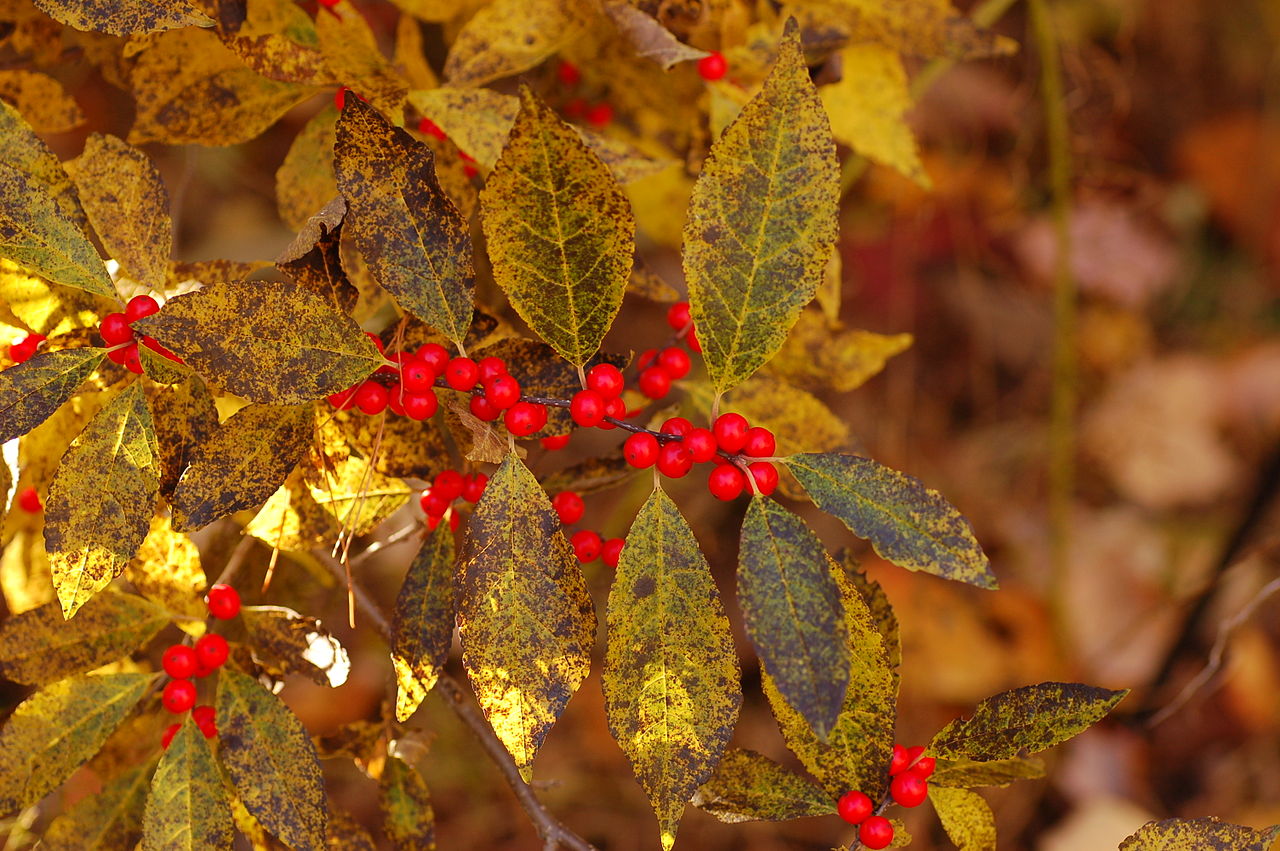The image captures the realistic close-up of a holly bush or a similar plant exhibiting signs of disease or decay. The focal point is the cluster of vibrant red berries adorning leaves that are multicolored and in various stages of discoloration—showing hues of yellow, green, brown, and almost black. The leaves are partially serrated and display noticeable aging or damage. The scene suggests an autumn setting, reinforced by blurred background details depicting other colored leaves, presumably on a forest floor. A subtle light filters in from the left side of the image, adding a touch of illumination to the otherwise somber and blurry surroundings.